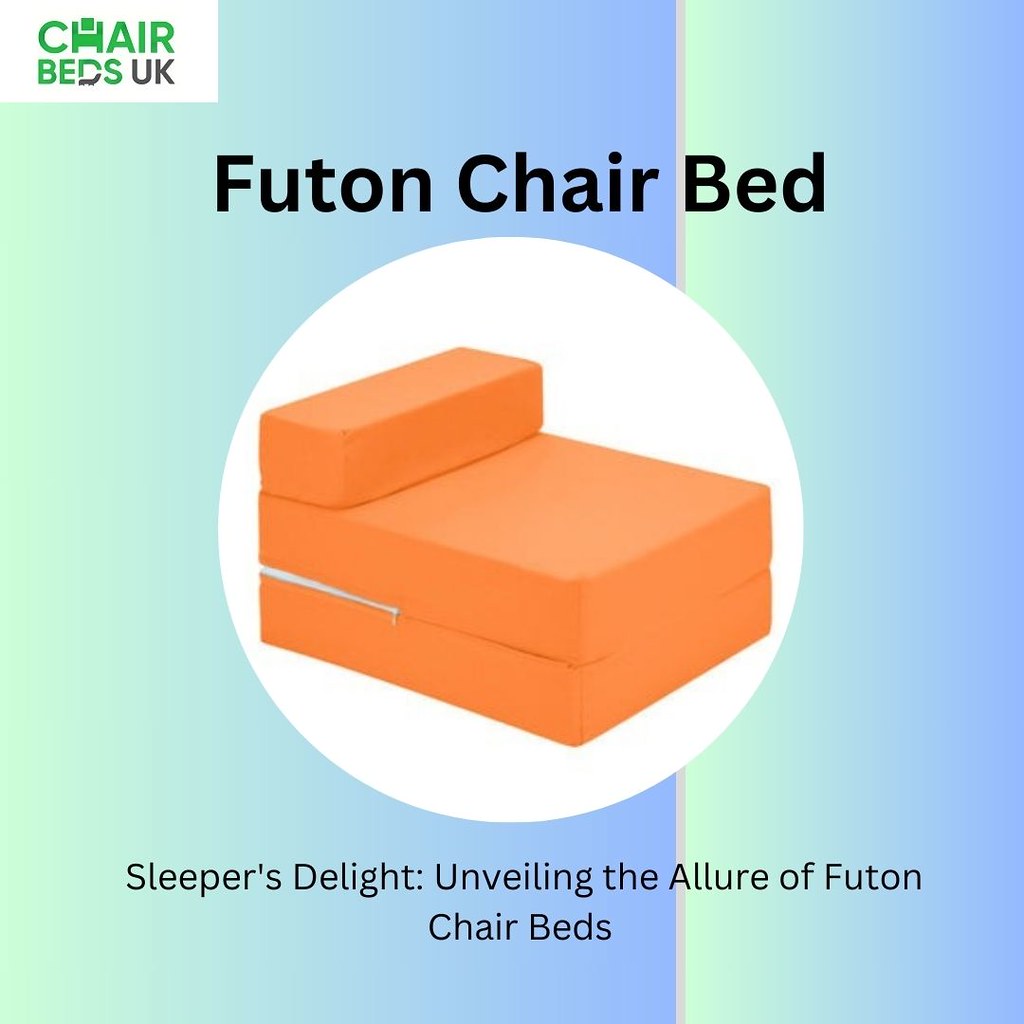This vibrant advertisement from the UK features a futon chair bed against a dynamic background composed of various shades of blue and green, blending seamlessly from darker blue on the left to lighter blue on the right. Central to the image is a white circle containing a detailed illustration of an orange futon chair bed. The top left corner of the image prominently displays the brand name "Chair Beds UK" in green with "UK" in black, alongside the company logo where the "H" is stylized as a chair bed. The text "futon chair bed" is written in black font directly above the central image. Beneath the graphic, the ad reads "Sleeper's Delight: Unveiling the allure of futon chair beds." The cushion on the futon chair bed appears to feature a zipper, adding to the detailed depiction of the product.